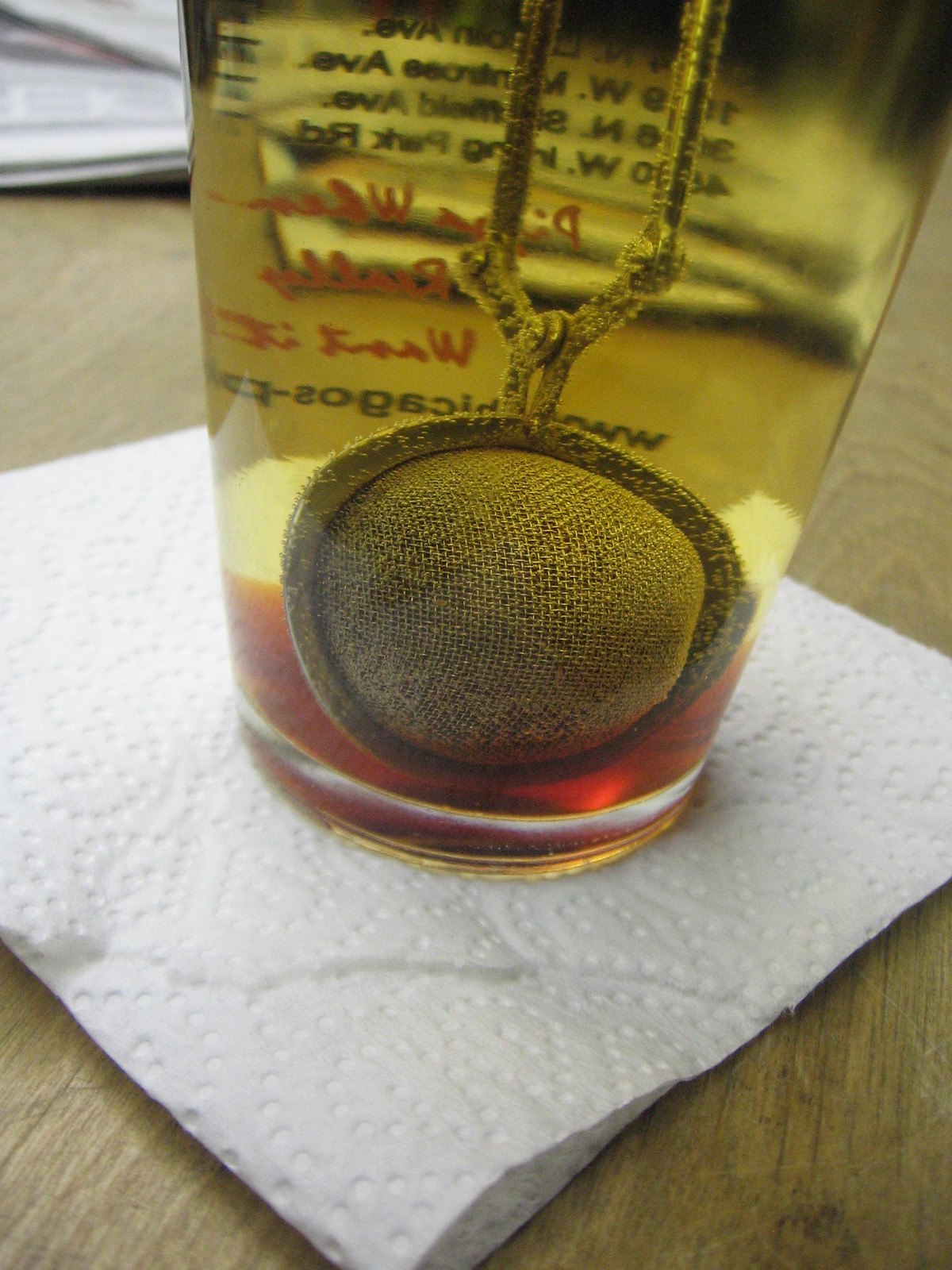The rectangular photograph captures a bottle or pint glass containing a yellowish clear liquid, which is steeping tea. This container is placed on a folded, white paper towel that showcases a bubble pattern, indicative of its absorption purposes, and rests on a wood grain table with visible fine lines and details. Through the glass, faint and unreadable black print, along with red scrolly writing, hints at possible business or promotional markings. The liquid inside the glass exhibits a gradient from a dark red or orange at the bottom to a murky green towards the top, suggesting a heavier concentration of substance at the base. Suspended within the liquid is a silver mesh tea infuser on a chain, giving the impression of a metal colander, with a round, mesh-like structure for steeping the tea leaves.